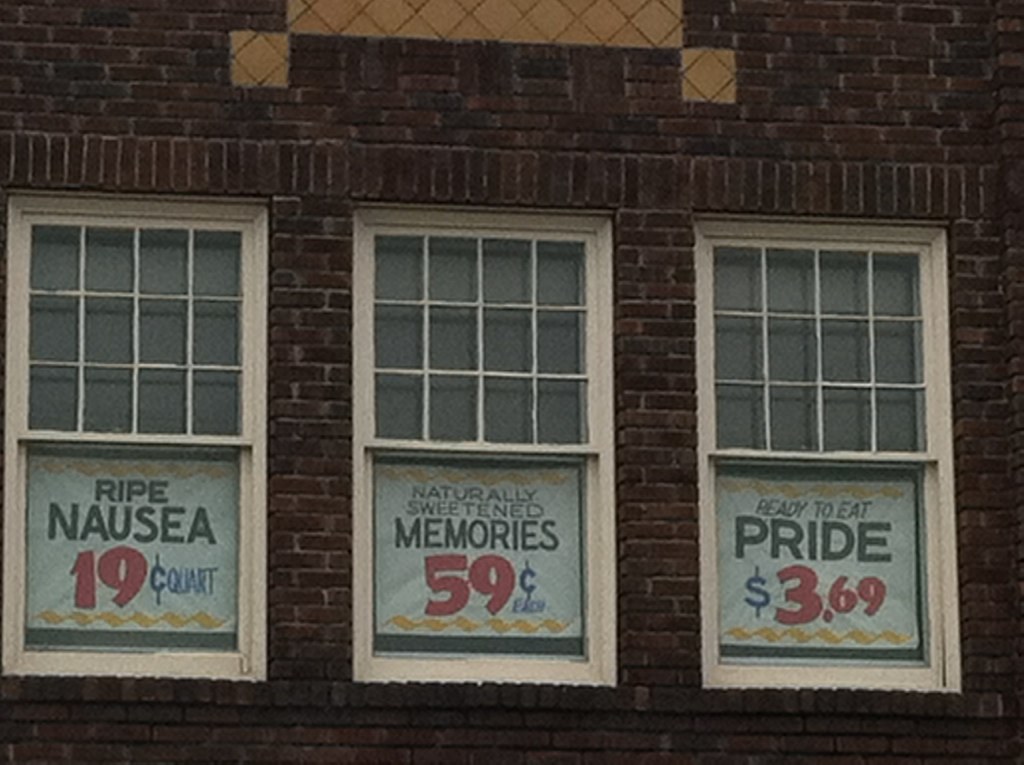This is a photograph of the side of an aged brick building, characterized by its gritty and dark ambiance, perhaps situated in an urban cityscape. The structure's brown bricks appear weathered and slightly dirty, adding to the overall vintage feel. Set into this brick facade are three white-framed windows with classic wood pane dividers. Each window features a peculiar ad in the bottom pane, mimicking old grocery produce signs but with a cynical twist. The window on the left promotes "Ripe Nausea" priced at 19 cents a quart, with the text divided into black, red, and dark blue colors. The middle window advertises "Naturally Sweetened Memories" for 59 cents each, also using a mix of black, red, and blue text. The rightmost window lists "Ready to Eat Pride" for $3.69, with the price highlighted in red. Below each price, a yellow-orange squiggle adds a graphic touch. Additionally, above the middle window is a decorative beige brick design set in a diamond pattern, with a single brick extending downward on either side of the window, emphasizing the central placement of this curious scene.